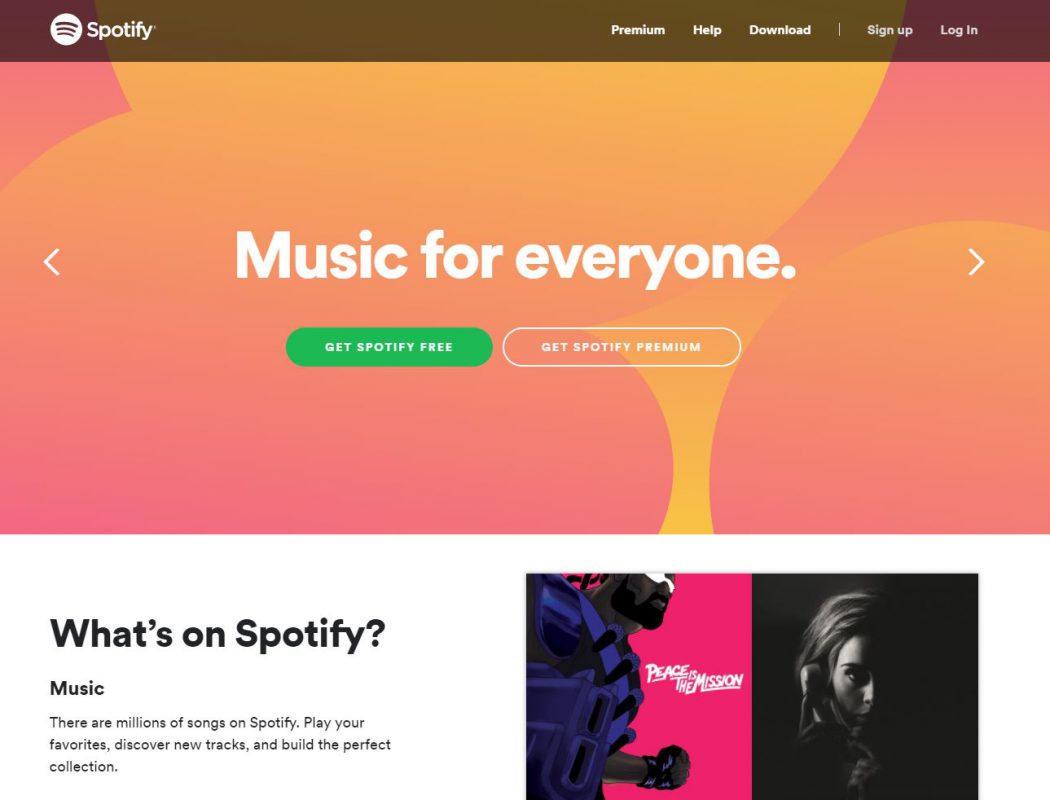This is an image of a Spotify advertisement featuring a prominent black bar across the top with "Spotify" in white lettering. Below this, options for "Premium," "Help," "Download," "Sign Up," and "Log In" are displayed. The main background is a gradient of orangish-pink hues embellished with a pattern of large and medium-sized circles.

The central message, "Music for everyone," is prominently written in white. Beneath this, a green circle reads "Get Spotify Free" in white lettering. Adjacent is another circle in a blend of orangish-pink and yellow shades that says "Get Spotify Premium," flanked by navigational arrows pointing left and right respectively.

In the bottom left corner, the text "What's on Spotify" is displayed in bold black lettering. Below this, the inscription "Music" explains, "There are millions of songs on Spotify. Play your favorites, discover new tracks, and build the perfect collection." Next to this text, a smaller section features two images: one of a person wearing a purple shirt and glasses, labelled "Peace Is The Mission," and another showing half of Adele's face. Adele is holding an old-fashioned telephone, with one hand pointing towards the earpiece and the other on the mouthpiece.